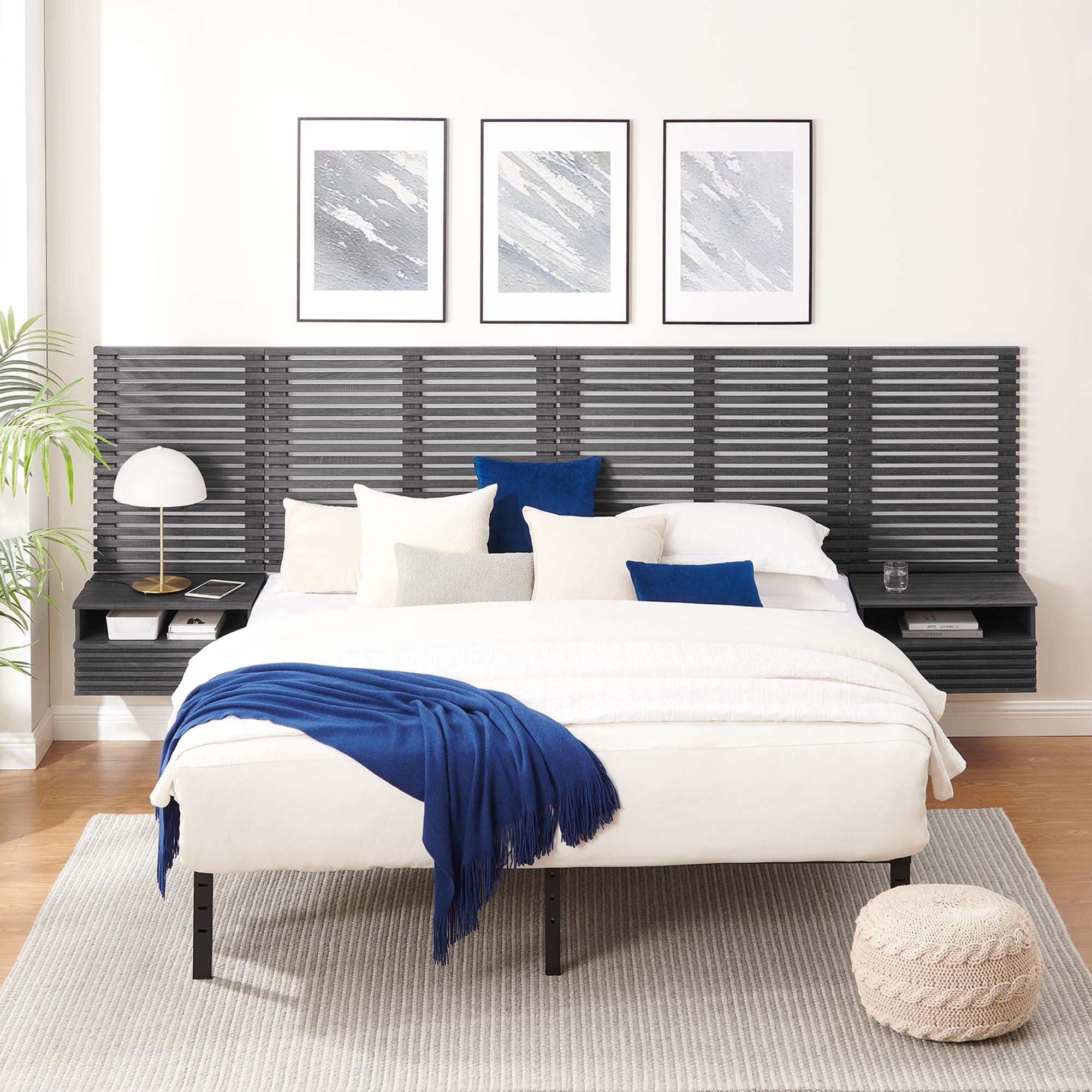This is a photograph of a very modern, serene bedroom centered around a white king-size bed with black legs. The bed is adorned with white linens, including a turned-down white comforter, white pillows for sleeping, and several throw pillows in white, medium blue, and a very light gray. A deep blue throw blanket is draped elegantly over the bottom left corner. The distinctive, integrated headboard features a black or dark gray slatted design, running horizontally to form floating nightstands on either side. These nightstands display a white lampshade with a lamp and a stack of books on the left, accompanied by a small plant. On the right nightstand, there is a glass of water and additional books. Above the headboard are three large, abstract prints in gray and white hues, matted in white and framed in black, adding to the minimalist aesthetic. The bed rests atop a grayish-white rug with light striping, on a hardwood floor, and is complemented at the foot by a white crocheted ottoman. The window light filtering through on the left side bathes the room in a soft glow, contributing to the tranquil, contemporary ambiance.